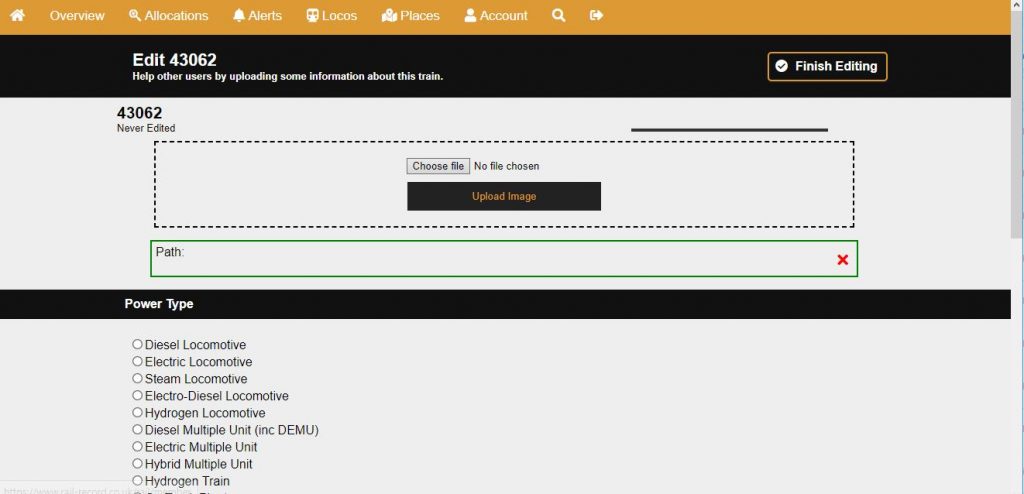The image showcases a detailed webpage interface of what appears to be a locomotive management or configuration platform. At the top of the page, a navigation toolbar is prominently displayed, featuring tabs labeled Overview, Allocations, Alerts, Logos, Places, and Account. Below this primary toolbar, the screen reads "Edit 43062," indicating the specific item or record currently being edited.

Beneath this header, there is an interactive toolbar designed for editing purposes, including a file path selector to upload images associated with the item. An extensive list of selectable options for different types of locomotives is presented under a “Power Type” dropdown menu. The available locomotive types include Electric Locomotive, Steam Locomotive, Electro-Diesel, Hydrogen Locomotive, Electrical Multiple Unit, Hybrid Multiple Unit, and Hydrogen Train, offering a wide range of customization for the user. 

The layout is well-organized, providing a streamlined experience for users to efficiently manage various locomotive configurations.